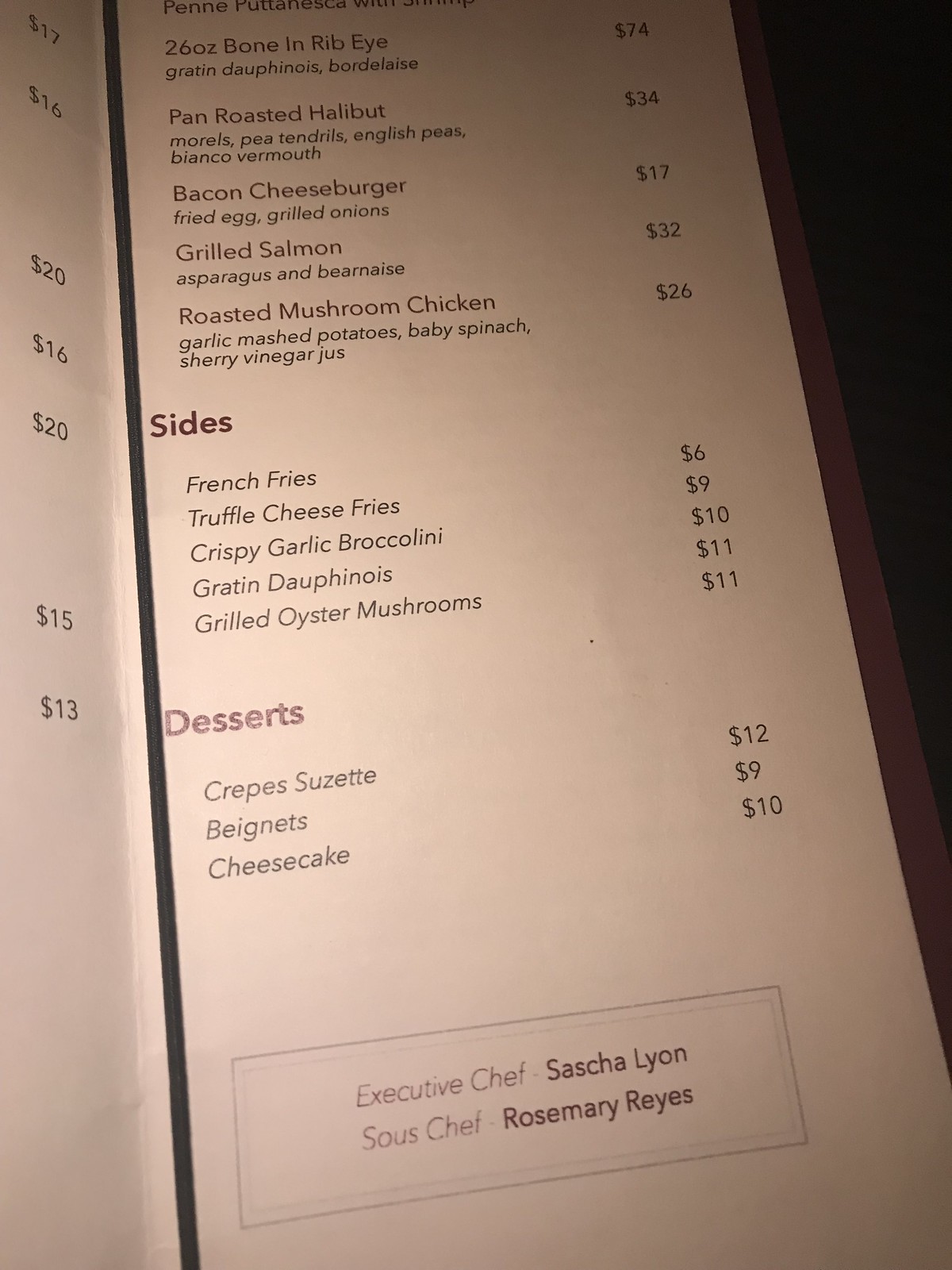The image depicts the right-hand side of a two-page restaurant menu, partially obscured by a triangular black area in the top upper right corner. The left side lists several prices: $16, $20, $16, $20, $15, and $13, although their corresponding dish descriptions are not visible.

On the visible right side, the menu details the following main courses and their prices: a 26-ounce bone-in ribeye for $24, a pan-roasted halibut possibly priced at $34, a bacon cheeseburger with fried egg and grilled onions for $12, grilled salmon for $32, and a roasted mushroom chicken served with garlic mashed potatoes, baby spinach, and a sherry vinegar jus for $26.

Additionally, the side dishes include french fries for $6, truffle cheese fries for $9, crispy garlic broccolini for $10, gratin dauphinoise for $11, and grilled oyster mushrooms for $11. The desserts feature crepe Suzette for $12, beignets for $9, and cheesecake for $10.

At the menu’s bottom, it credits the executive chef, Sasha Lyon, and the sous chef, Rosemary Reyes.